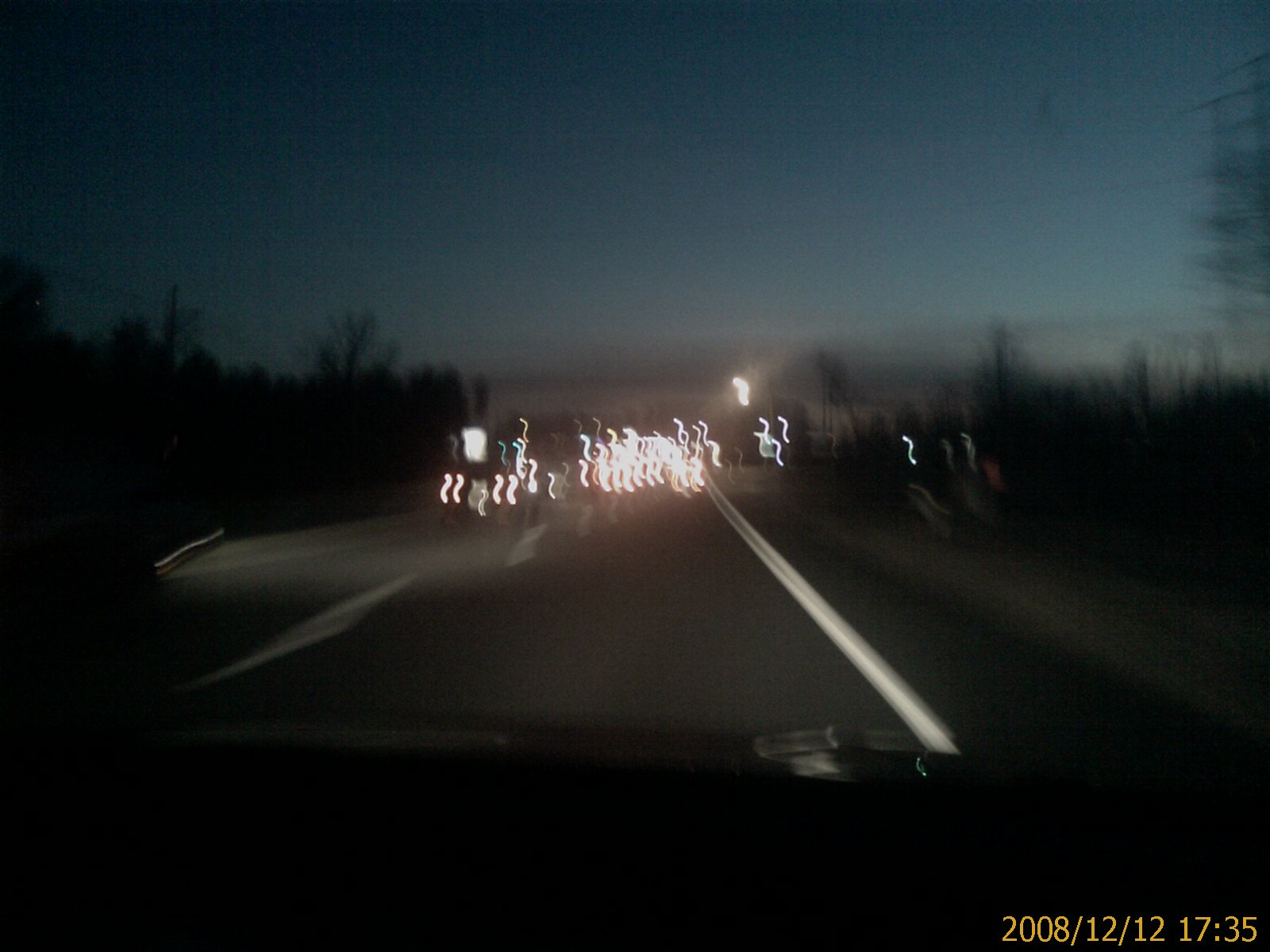A blurry, dimly lit nighttime photo captures the view from a car's windshield as it travels down a road. Straight ahead, squiggly blurred headlights of other vehicles form a stream of lights that extend into the distance. The road's lane disappears towards a faintly illuminated horizon, with a subtle glow under a dark blue sky. Off to either side of the road, the silhouettes of tall, dark trees are just visible. In the lower right corner of the photo, a date stamp reads "2008 2012 1735," and a small portion of the car's dashboard can be seen at the bottom edge of the image.